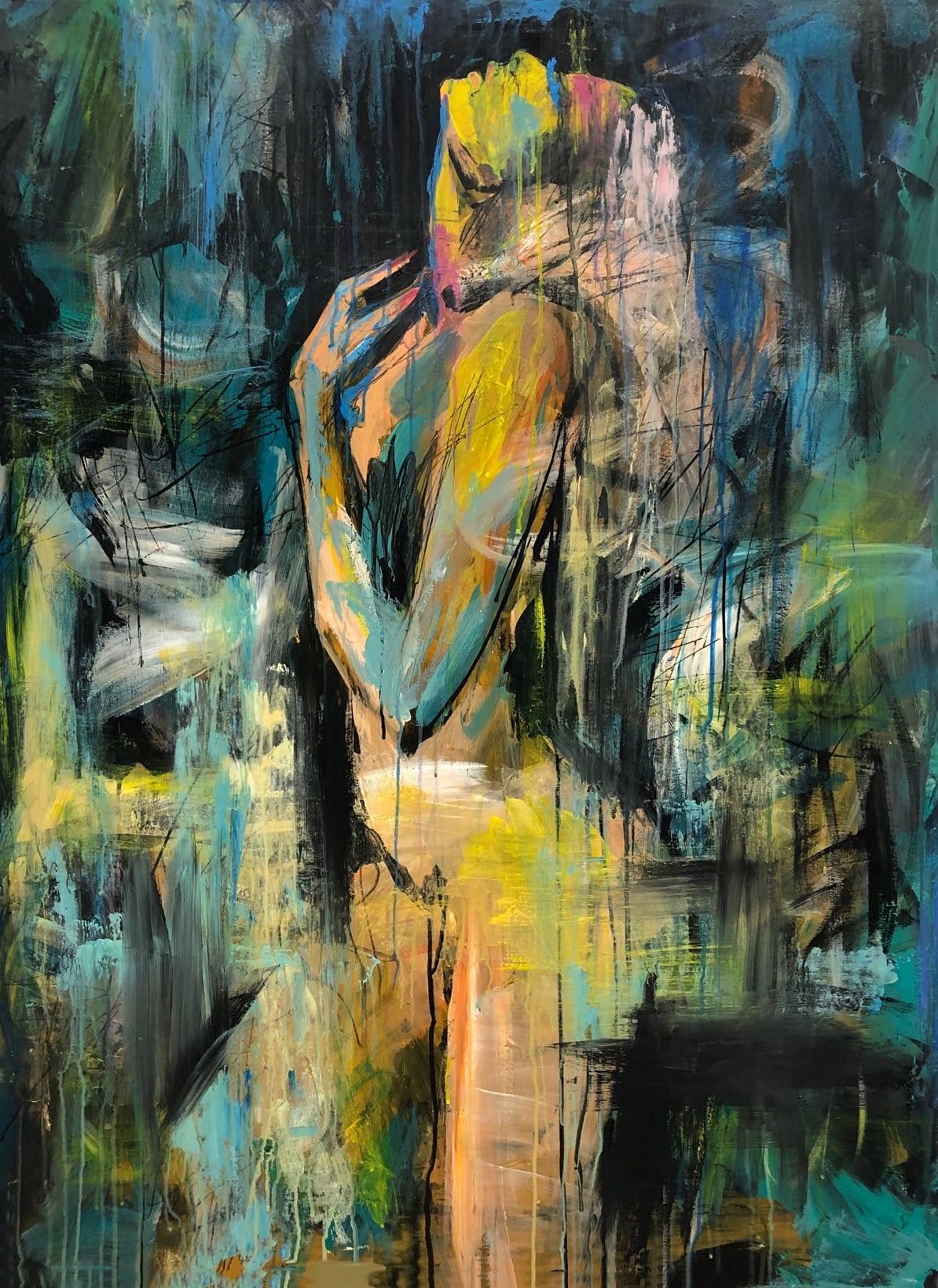This abstract painting portrays the side view of a woman facing left, set against a vibrant background of black, blue, white, green, and yellow hues, with additional splashes of light blue, dark blue, orange, teal, pink, and purple. The woman features striking yellow hair with a pink section at the back. Her left hand is raised, almost touching her face, while her left hand rests on her chest, suggesting a pose that highlights her bending arm and leg. 

She predominantly appears in yellow and pink tones, with broad strokes implying the use of either a palette knife or a very large brush. Notably, her eyelashes are depicted in blue and her eyebrows in reddish tones. The image is somewhat fragmented and abstract, though the central figure and her form are discernible. Additional details include potential white clothing covering the lower part of her body. The composition is framed at the bottom right with a horizontal and vertical black line forming a right angle, adding a geometric element to the painting.